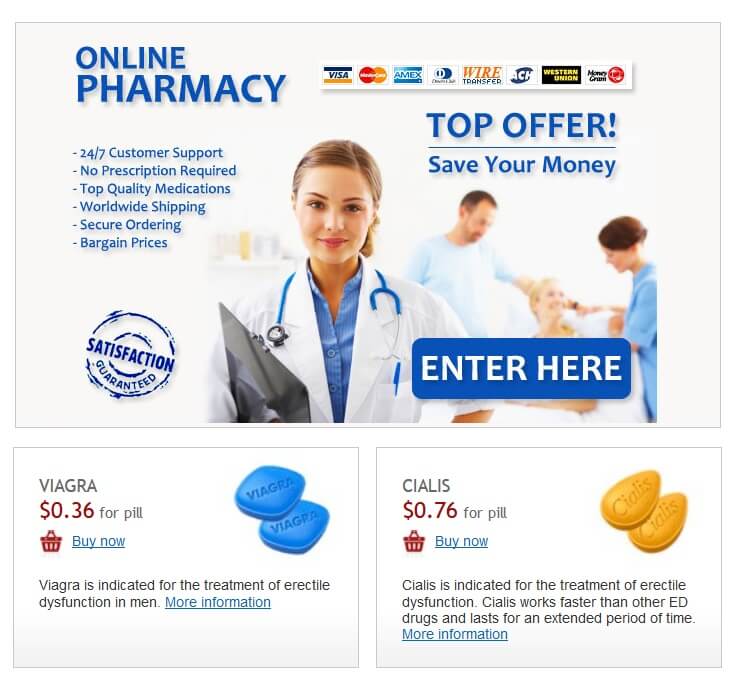This screenshot displays a website sorted into three distinct sections, all enclosed by thin gray borders. The top section boasts a header with the phrase "Top Offer, Save Your Money" followed by a promotional panel. It features a smiling female doctor in a white lab coat with a blue stethoscope draped around her neck and a blue button-up shirt. She clutches a clipboard in her right hand. Blurred in the background, a patient interacts with two other medical professionals. The top left corner of this section highlights the title "Online Pharmacy" in bold blue text, accompanied by various payment method icons. Below this, it lists key selling points: "24-7 Customer Support," "No Prescription Required," "Top Quality Medications," "Worldwide Shipping," "Secure Ordering," and "Bargain Prices." A "Satisfaction Guaranteed" blue stamp is prominently displayed beneath these points, followed by a large blue button reading "Enter Here" in white text.

The lower half of the image is divided into two horizontal boxes. The left box advertises "Viagra" for 36 cents per pill, accompanied by an image of two blue Viagra tablets and a "Buy Now" button. Brief descriptive text follows this advertisement. The right box promotes "Cialis" at a price of 76 cents per pill, illustrated with two yellow Cialis pills and accompanied by similar descriptive text.